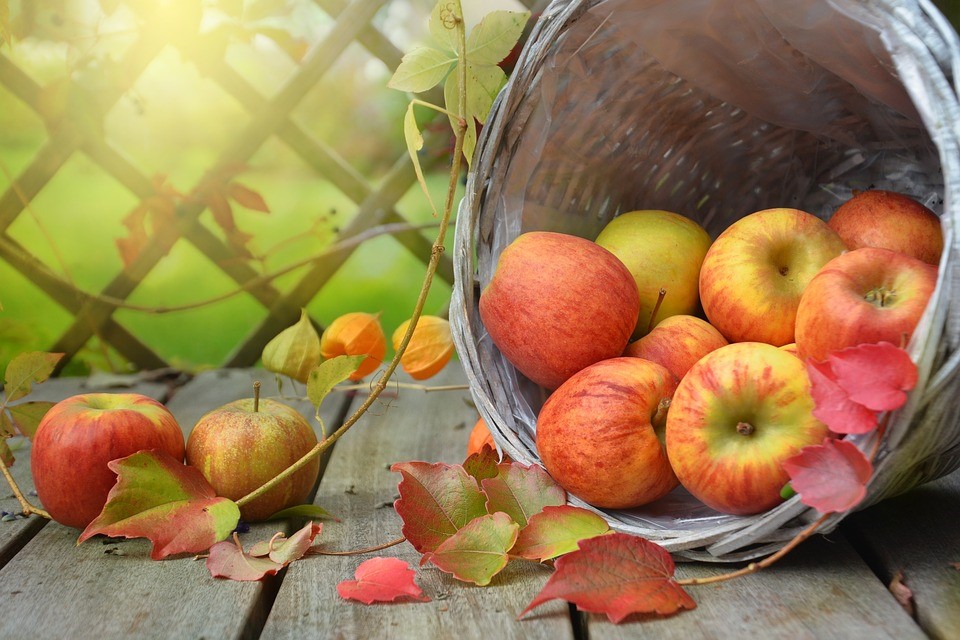The photo depicts a scenic autumn scene with a wicker basket of apples tipped over on a wooden deck. The deck's wooden slats are visible, with about four planks discernible. The apples, a mix of red, green, and yellowish hues, spill out of the basket, some remaining inside while two larger apples rest on the deck next to it—one predominantly red and the other red and green. Scattered around the apples are leaves, adding to the seasonal feel. Behind the scene, a wooden lattice fence adorned with foliage and vines filters through a glimmer of sunlight, with a patch of vivid green grass peeking through in the background. The overall color palette of the photo includes rich reds, greens, yellows, browns, and tans, contributing to a warm, rustic ambiance.